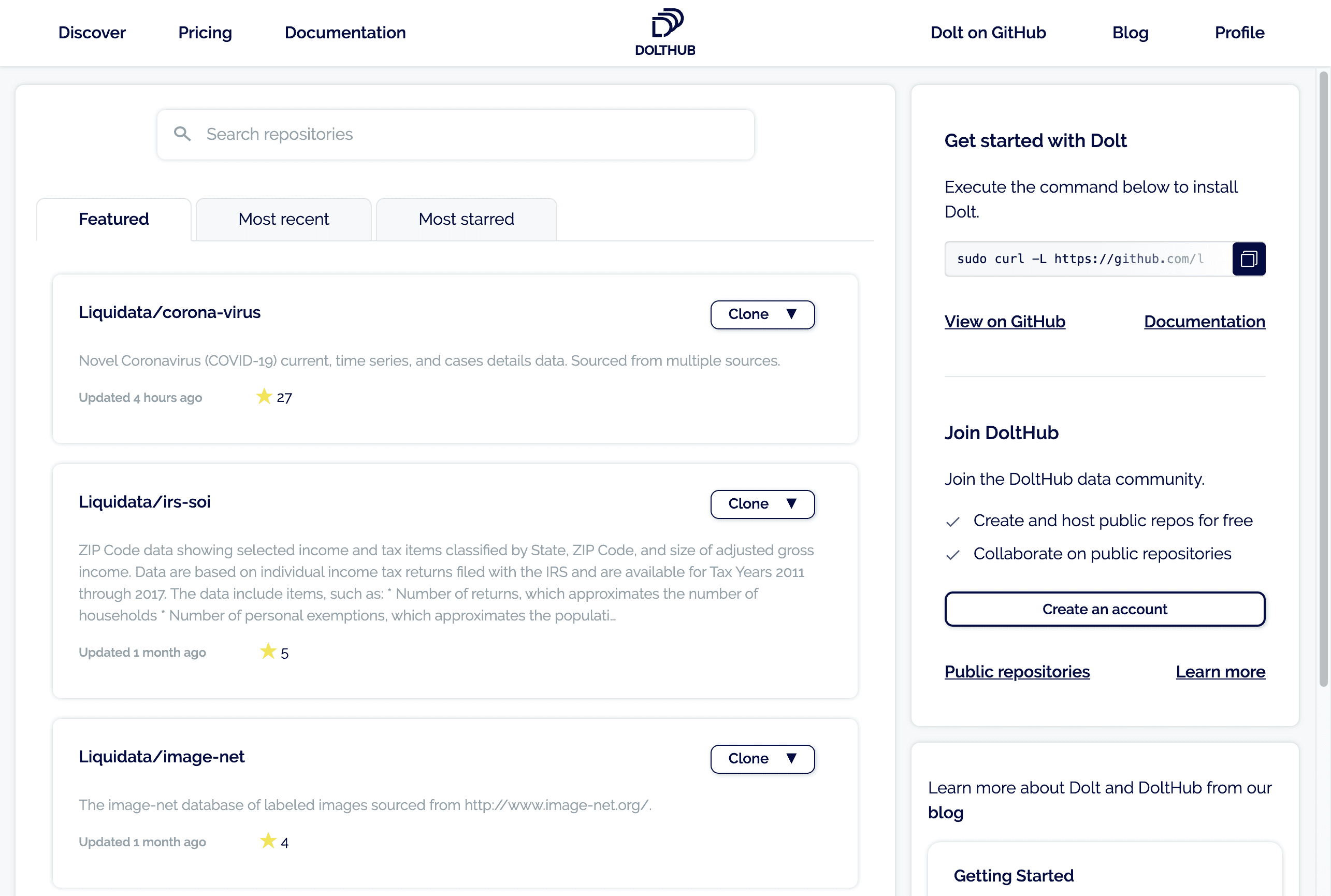The image features a predominantly white background with several distinct elements arranged across it. At the top, from left to right in black text, it reads "Discover Pricing Documentation." Centered below this is a black logo resembling an uppercase letter "D," followed by the text "DOLTHUB."

Beneath "DOLTHUB," there are navigation links reading "Do it on GitHub," "Blog," and "Profile." On the right side of this header, there is a section titled "Get Started with DOLTH" with instructions to execute a command for installing DOLTH, followed by a URL link. Additionally, there are links labelled "View on GitHub" and "Documentation."

Further down, the text encourages users to "Join on DoItHub - Join the DoItHub data community," emphasizing the ability to "Create and host public repos for free" and "Collaborate on public repositories." A prominent button labeled "Create Account" is followed by links to "Public Repositories" and "Learn More." The next section elaborates with "Learn More about DoIt and DoItHub from our blog," and under it, "Getting Started."

On the left side, there is also a white background at the top, featuring a search bar labeled "Search Repositories." Below the search bar are three tabs: "Featured," "Most Recent," and "Most Starred," with the "Featured" tab currently selected. Under the "Featured" tab, three sections are listed: "Liquidata/Coronavirus," "Liquidata/IRSSOI," and "Liquidata/Image-Net."